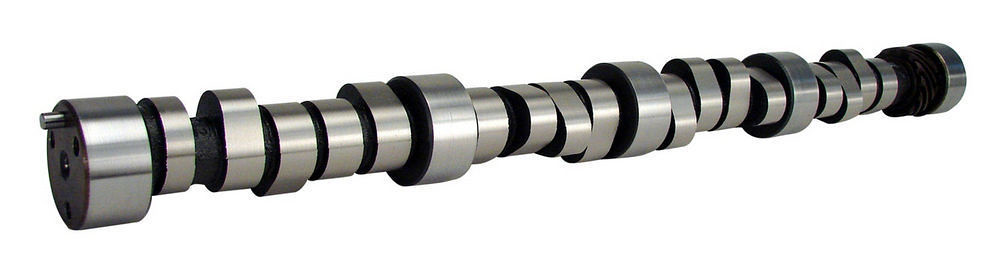In this image, we see an automotive part—essentially a long silver cylinder with wider ends positioned horizontally against a white background. The cylinder is adorned with 22 circular elements that appear to be evenly distributed along its length. These elements are predominantly silver and black, with variations in shape including both round and egg-shaped forms. One of these elements stands out by being entirely black. Each element features black tops and bottoms with silver ridges encircling the sides, with some elements appearing more flat due to their orientation. The context suggests the image might be used in a magazine or an online advertisement to showcase the product, with no accompanying text. The background is plain white, adding focus to the detailed metallic structure of the part.